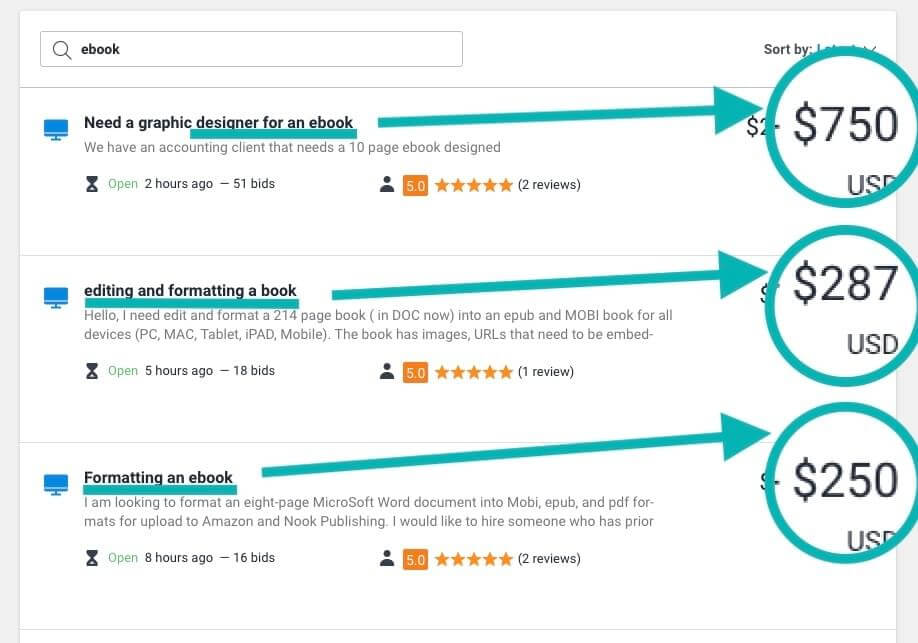In this image, a search box is displayed with the search term "e-book" entered in the top left corner, resulting in three detailed listings. 

1. The first listing is titled "Meet a Graphic Designer for an E-Book," detailing a project for an accounting client who requires a 10-page e-book design. This listing was posted two hours ago, has received 51 bids, and boasts a 5-star rating with 2 reviews. Notably, the ratings are highlighted in orange. The price for this project, $750 USD, is emphasized with a green underline and circled in green to draw attention.

2. The second listing, "Editing and Formatting a Book," describes the need for editing and formatting a 214-page book now in .doc format, converting it to EPUB and MobiBook formats for compatibility across all devices, including PC, Mac, tablets, iPads, and mobiles. The project description mentions the inclusion of images and embedded URLs, stressing the requirement for comprehensive formatting. This listing was posted five hours ago, has attracted 18 bids, and also features a 5-star rating with 1 review. The price is $287 USD, highlighted with a blue underline and black font, and circled for emphasis.

3. The third listing, titled "Formatting an E-Book," involves formatting an 8-page Microsoft Word document into Mobi, EPUB, and PDF formats for upload to Amazon and Nook Publishing. The client is specifically seeking someone with prior experience. This listing, posted eight hours ago, has garnered 13 bids and maintains a 5-star rating with 2 reviews. The price for this project is listed as $250 USD and is indicated with a dark green underline and a circled price for easy visibility.

Each listing is meticulously detailed, showcasing the variety of e-book related tasks up for bidding, along with their respective posting times, number of bids, ratings, and prices.